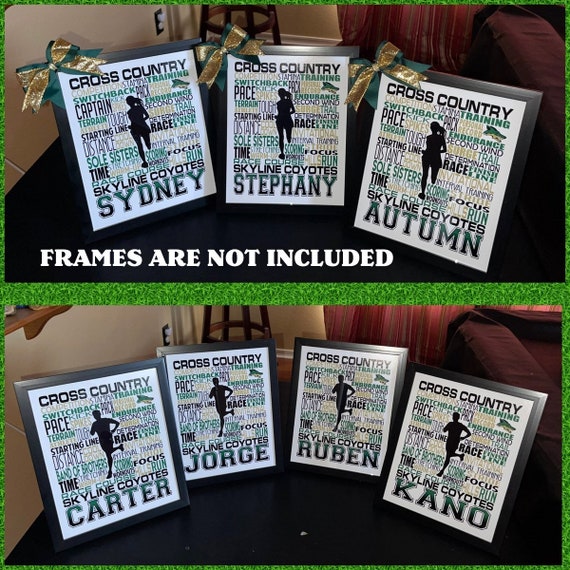The image showcases two pictures set against a green background, likely an advertisement for personalized cross-country awards. The top picture features three framed awards with green and gold bows on the top left corner. Each frame contains a stylish text map centered around a silhouette of a girl running. The text includes cross-country-related terms like "competitions," "training," "switchback," "pace," "spikes," "distance," "time," and "focus." The top of each paper reads "Cross Country," with the bottom displaying "Skyline Coyotes" and individual names—Sydney, Stephanie, and Autumn—in large green letters. Notably, there's an overlay text stating "frames are not included." 

The bottom picture presents four similar awards aimed at boys, each featuring the silhouette of a boy running. These also exhibit the "Cross Country" theme and contain terms related to the sport. Below the "Skyline Coyotes" text, the names Carter, George, Ruben, and Kano are prominently displayed. These awards are designed to be personalized for the athletes, making them perfect keepsakes to honor their achievements in cross-country running.